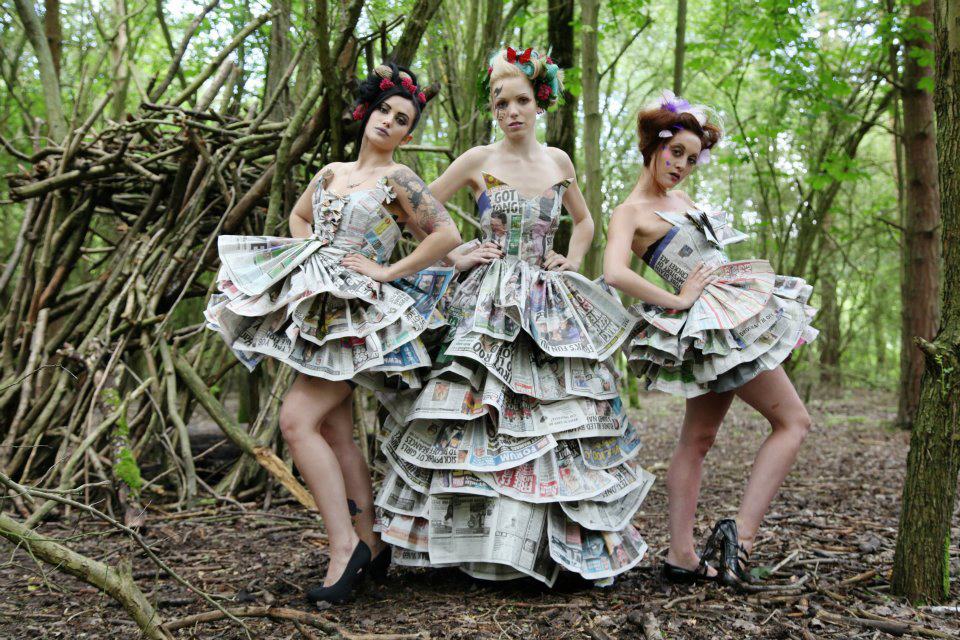In this captivating photograph, three women stand on a wood-chipped pathway amidst a sunlit forest, with a thicket of trees and a rustic structure of woven branches in the background. Each woman is attired in a striking dress crafted from brightly colored newspaper, featuring hues such as purple, red, and blue. On the left, the woman dons a short, strapless dress with three layers of ruffled paper, while the woman in the middle wears a similar newspaper dress with ruffles cascading to the ground. The woman on the right mirrors the left in a short, ruffled, strapless dress. All three have their hands confidently placed on their waists, their expressions serious and unsmiling. Their hair is styled in exaggerated, poofy buns adorned with colorful objects, including red butterflies and vibrant ribbons, matching their overdone and vividly colored makeup. The forest around them is scattered with dry leaves and twigs, allowing ample light to filter through the trees, creating a surreal and whimsical setting for this unconventional fashion statement.